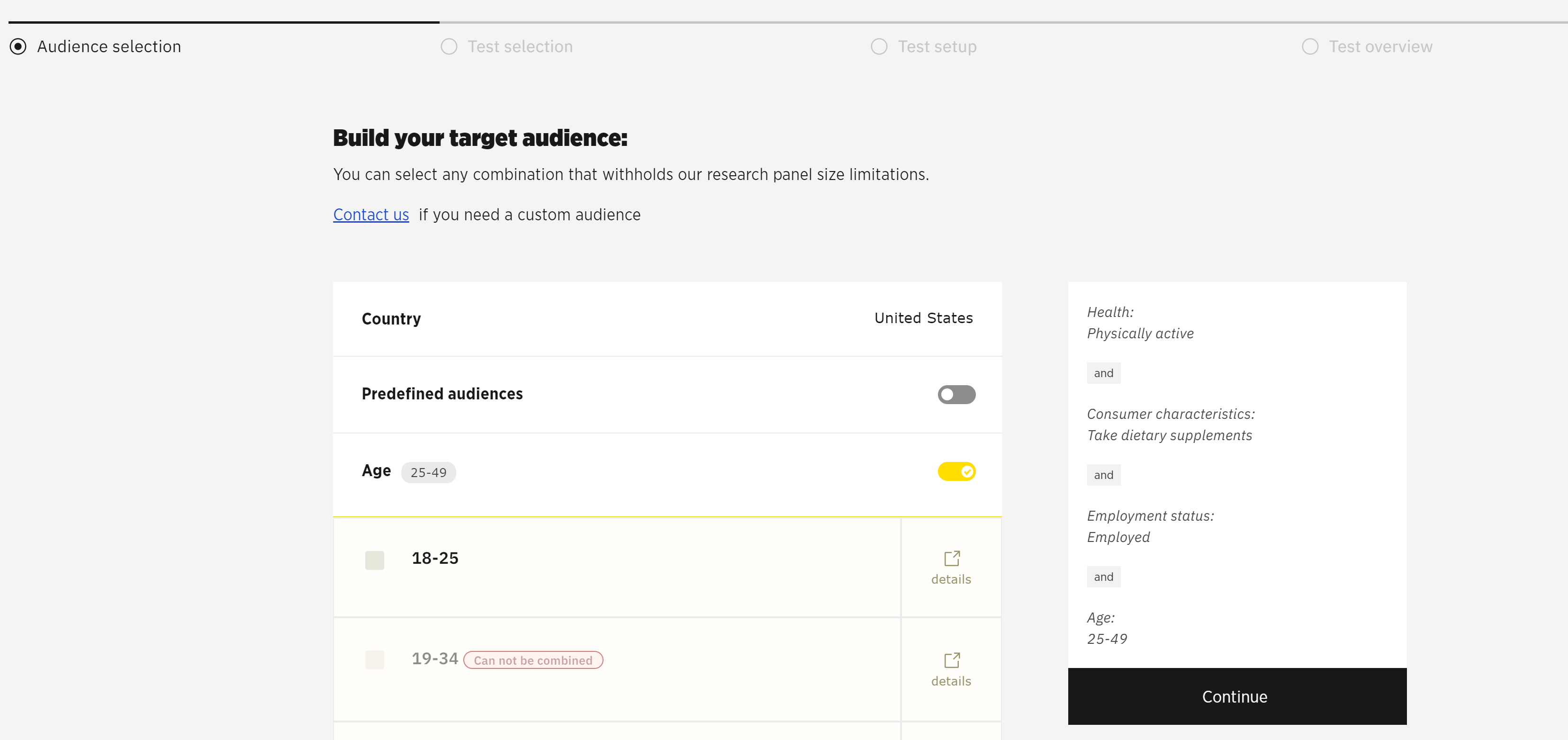The screenshot appears to be from a user interface of an audience selection tool, with a clean gray background and two white rectangular sections. At the top of the screenshot, the title "Audience Selection" is prominently displayed, with a radio button next to it that indicates it has been selected. Various sections follow, including "Test Selection," "Test Setup," and "Test Overview."

The main instructions suggest: "Build your target audience. You can select any combination that complies with our research panel size limitations. Contact us if you need a custom audience." Below this, the user can specify parameters for the target audience.

The geographical selection is set to the "United States." The option for predefined audiences is available but currently turned off. Age parameters are specified, with the age range 25 to 49 being active (slider on), though the ages 18 to 25 and 19 to 34 cannot be combined. Additional characteristics include:
- **Health**: Physically active.
- **Consumer Characteristics**: Takes dietary supplements.
- **Employment Status**: Employed.
  
The image is wide in orientation with no photographic elements. It contains no depictions of people, animals, birds, plants, flowers, trees, buildings, vehicles, or any form of aerial transportation such as airplanes or helicopters.